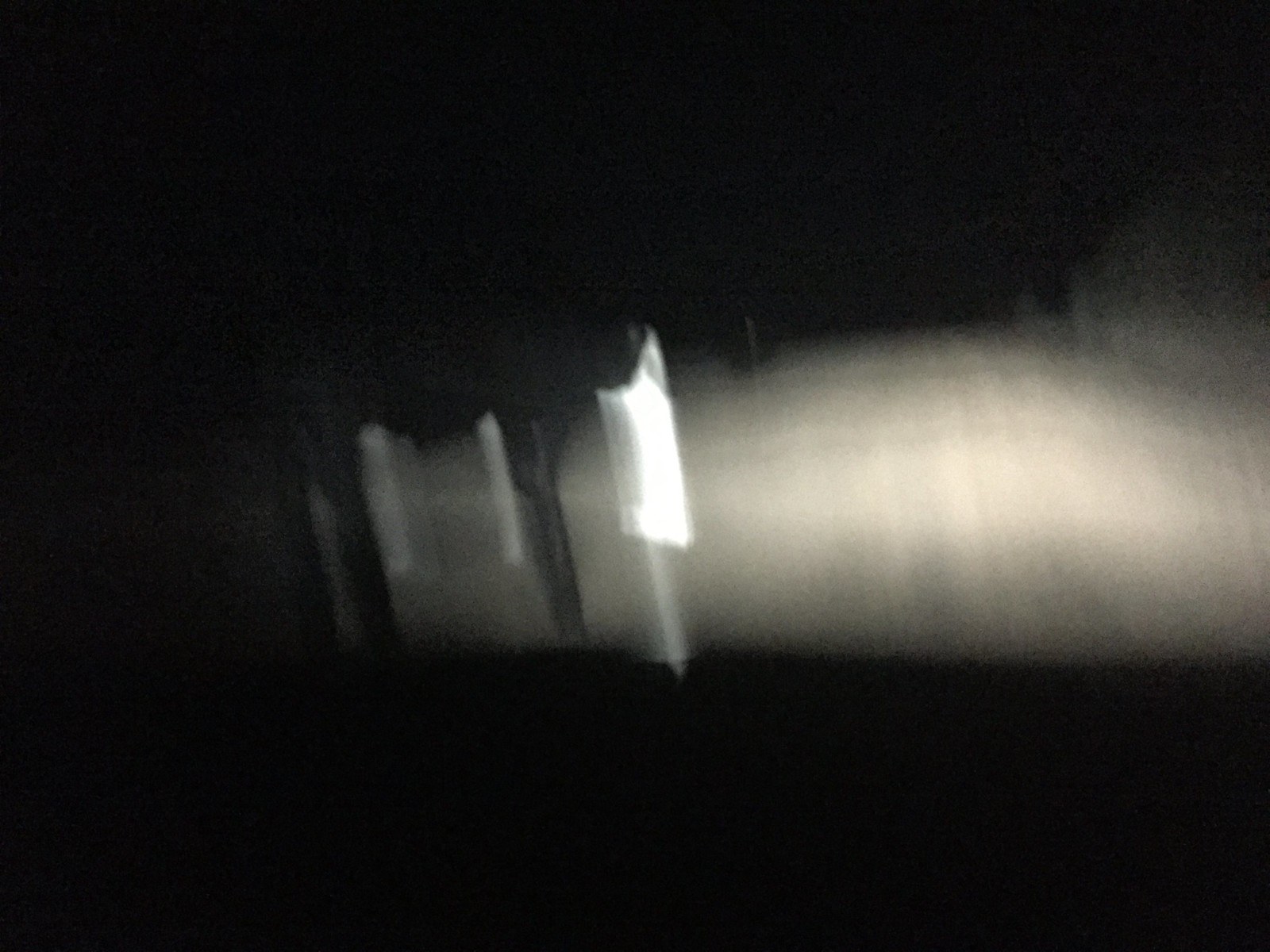The photo features a predominantly dark background with an enigmatic interplay of light and shadow. The top and bottom portions are shrouded in blackness, separated by a light blur that gradually brightens towards the right side of the image. Dominating the left side is a gray blob streaked vertically by stark black and white lines. Intriguingly, a sharp-edged white rectangular piece emerges in the middle of the photo, acting as a focal point. This central light source casts a striking glare, creating an impression of sunlight hitting the right side of the blob. Accentuating the composition, a bright highlight in the center glows intensely, extending from a quarter of the way from the left to the far right, with a hazy yellow light subtly creeping in from the right. The image exudes an ethereal quality, where forms and lines intermingle in a scene both abstract and evocative.